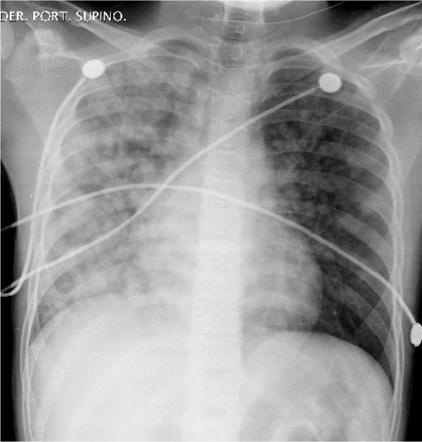The photograph is a detailed black and white x-ray of a human torso, taken from the chin down to about mid-belly. The background is predominantly black, accentuating the semi-transparent white shades that highlight the captured anatomy. The primary focus is on the skeletal structure, showcasing a clear view of the ribcage, spine, shoulder blades, neck bones, and collarbones. Additionally, the x-ray reveals partial outlines of various internal organs. Notably, there are three circular electrodes attached: one on each shoulder and one on the right side of the waist, all connected by white wires extending towards the left. In the top left corner, there's white text imposed on the image that reads "DER.PORT.SUPINO." The x-ray's crisp representation of the bones and misty shading of the soft tissues provides a classic radiographic visual of the human torso.